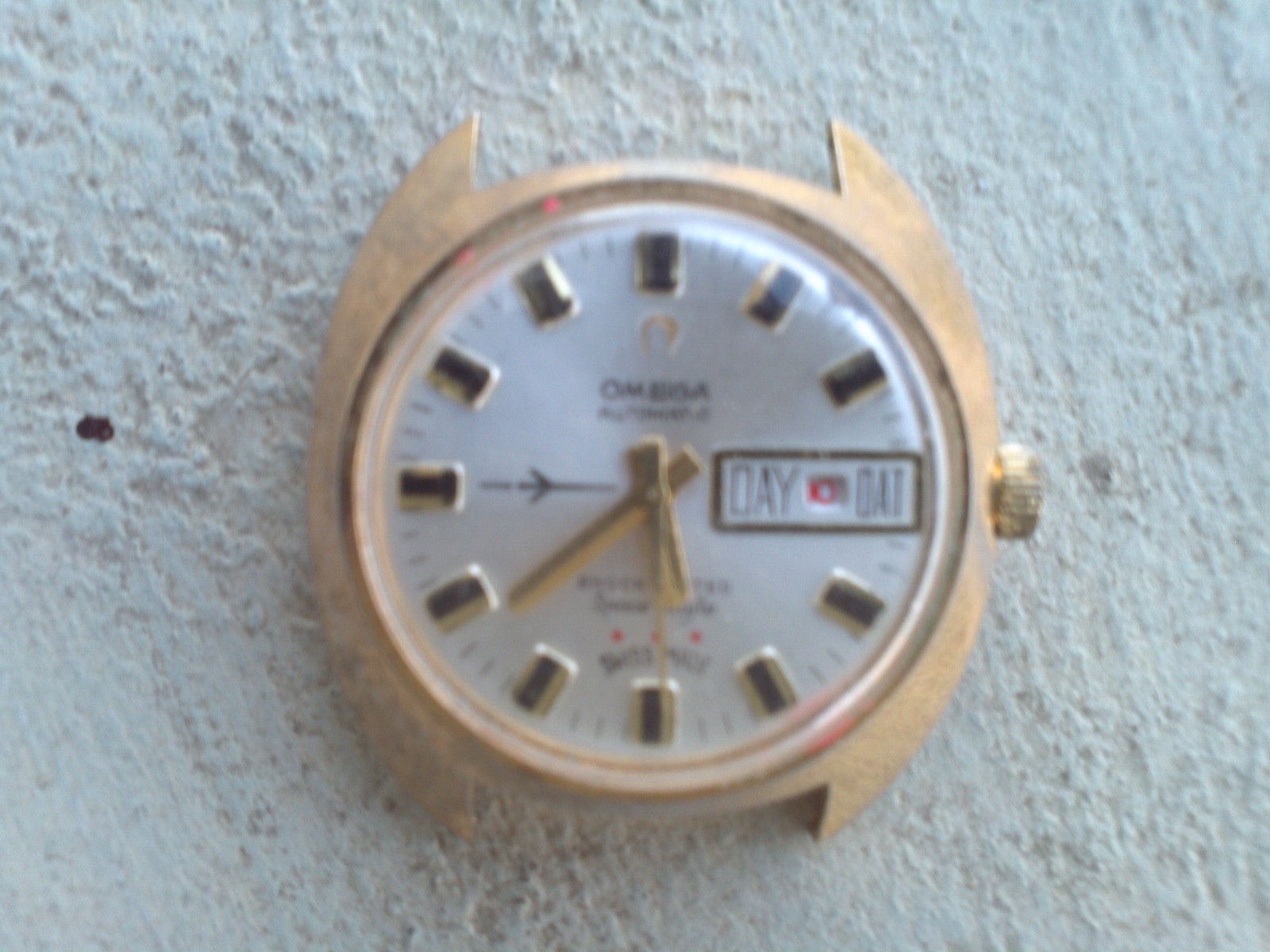The image features a zoomed-in, detailed close-up of a vintage Omega watch face, set against a rough, off-white, concrete-like surface. The watch is gold with no visible band, revealing the open spots where the band would attach. The face is primarily white, adorned with black stones at each hour mark, each bordered in gold, and smaller white lines marking the minutes. 

The words "Omega" are prominently displayed at the top of the face. The watch also features gold minute, hour, and second hands and a day marker. The watch hands indicate that it is stopped at 5:39 and 30 seconds. At the bottom, there are faint indications of text likely reading "Swiss Made." The overall impression is of an older, possibly tarnished gold timepiece with intricate detailing, indicative of its vintage Swiss craftsmanship.